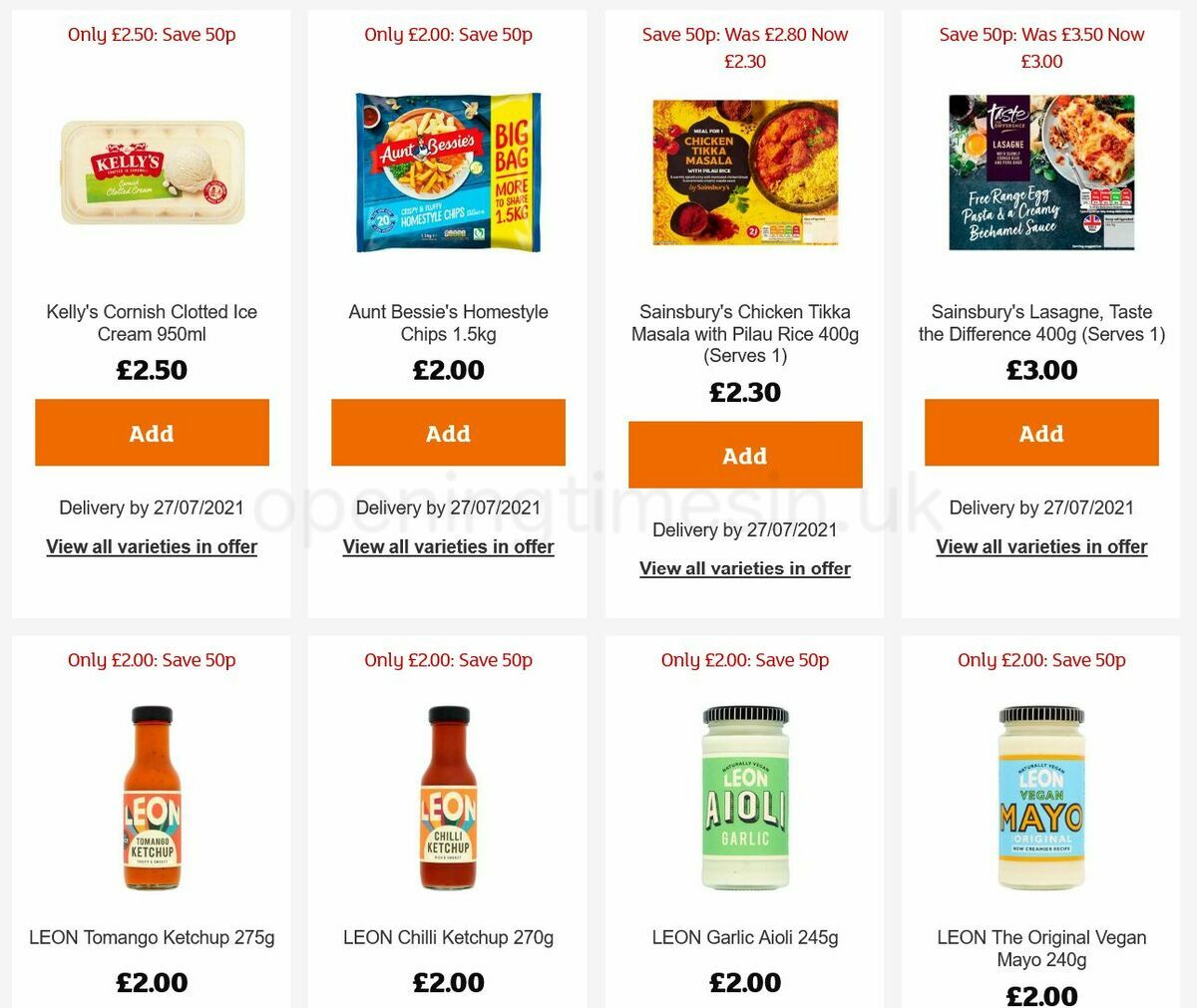The webpage displays a grocery shopping interface set against a light gray background. Each product is presented in individual white rectangular boxes accented with black text. Some text elements, particularly those highlighting actions or prices, feature a blend of orange and red colors, adding a pop of visual emphasis.

The layout includes four distinct products per row, arranged in two neat rows. Each product box contains the item's name, price, and an "Add" button situated underneath. However, the "Add" buttons, styled in orange with white text, are fully visible only in the top row and partially cut off in the second row.

Prominent at the top of the display, there is an announcement for delivery by July 27, 2021. Featured products include Kelly's Cornish Clotted Ice Cream, Aunt Bessie's Homestyle Chips, Sainsbury's Chicken Tikka Masala with Pilau Rice, and Sainsbury's Lasagna from the "Taste the Difference" range. The assortment also showcases various ketchup and mayo-based sauces.

Additionally, there are orange links with white text in the top row, inviting customers to "View all varieties in the offer," providing a gateway to explore more product options within the same category.